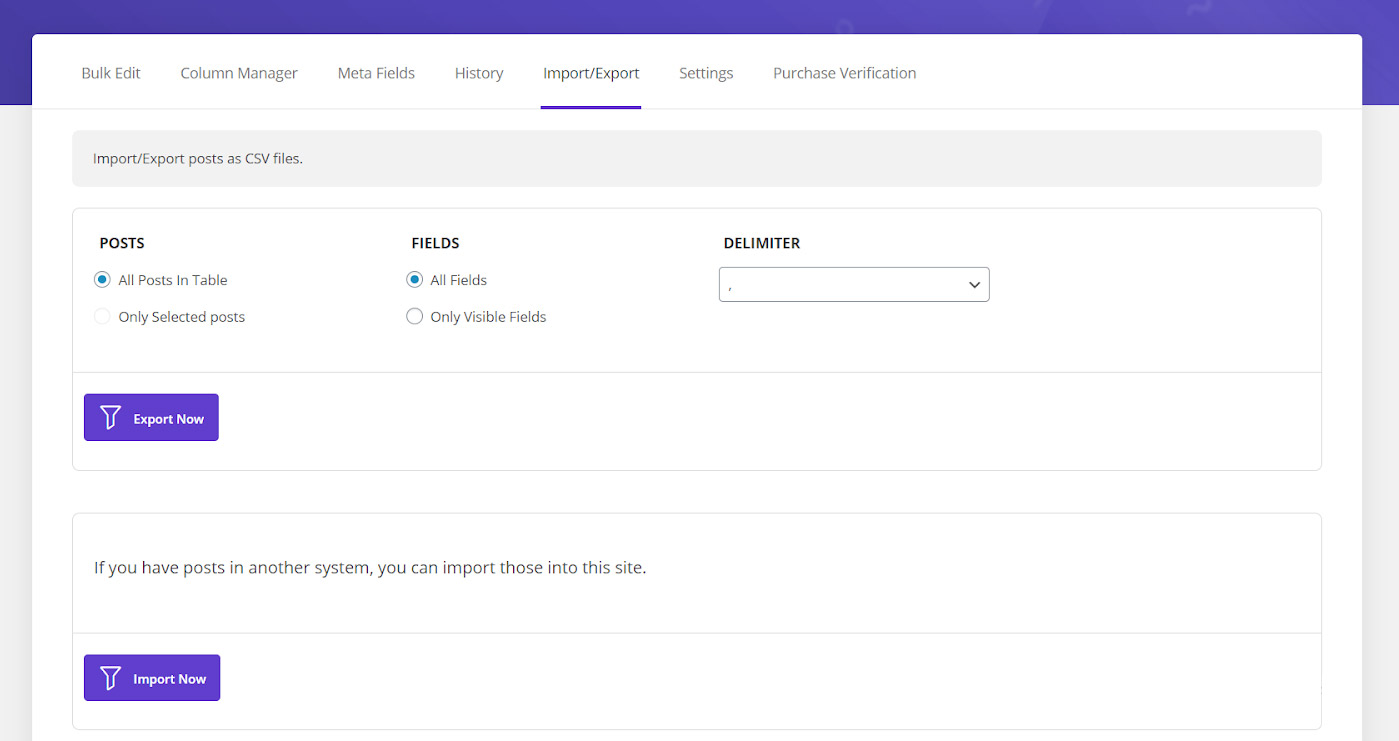### Caption:

The image displays a main menu interface with a blue header at the top. Below the header, a pop-out menu lists several options, with most of them grayed out: Bulk Edit, Column Manager, Metafields, History, Import, Export, Settings, and Purchase Verification. Only the 'Import' and 'Export' options are active, highlighted in black with a blue underline.

Underneath the menu, a gray horizontal line spans the width of the screen, labeled "Import Export." Below this, a gray boxed section explains the functionality: "Import Export posts as CSV files." Within this section, there's a lined-out, gray field with options for exporting posts. The options include "All posts in table" and "Only selected posts," with "All posts in table" currently selected.

Next, the interface provides choices for "Fields," offering "All fields" and "Only visible fields," with "All fields" chosen. A drop-down menu for selecting a delimiter is visible but currently unselected. A blue button labeled "Export Now" is situated beneath these options.

Further down, another gray-lined boxed section provides import functionality details: "If you have posts in another system, you can import them into this site." Below this message, there's a blue button labeled "Import Now." The background of the interface is predominantly white, with thin gray margins on each side, maintaining a clean and simple layout.